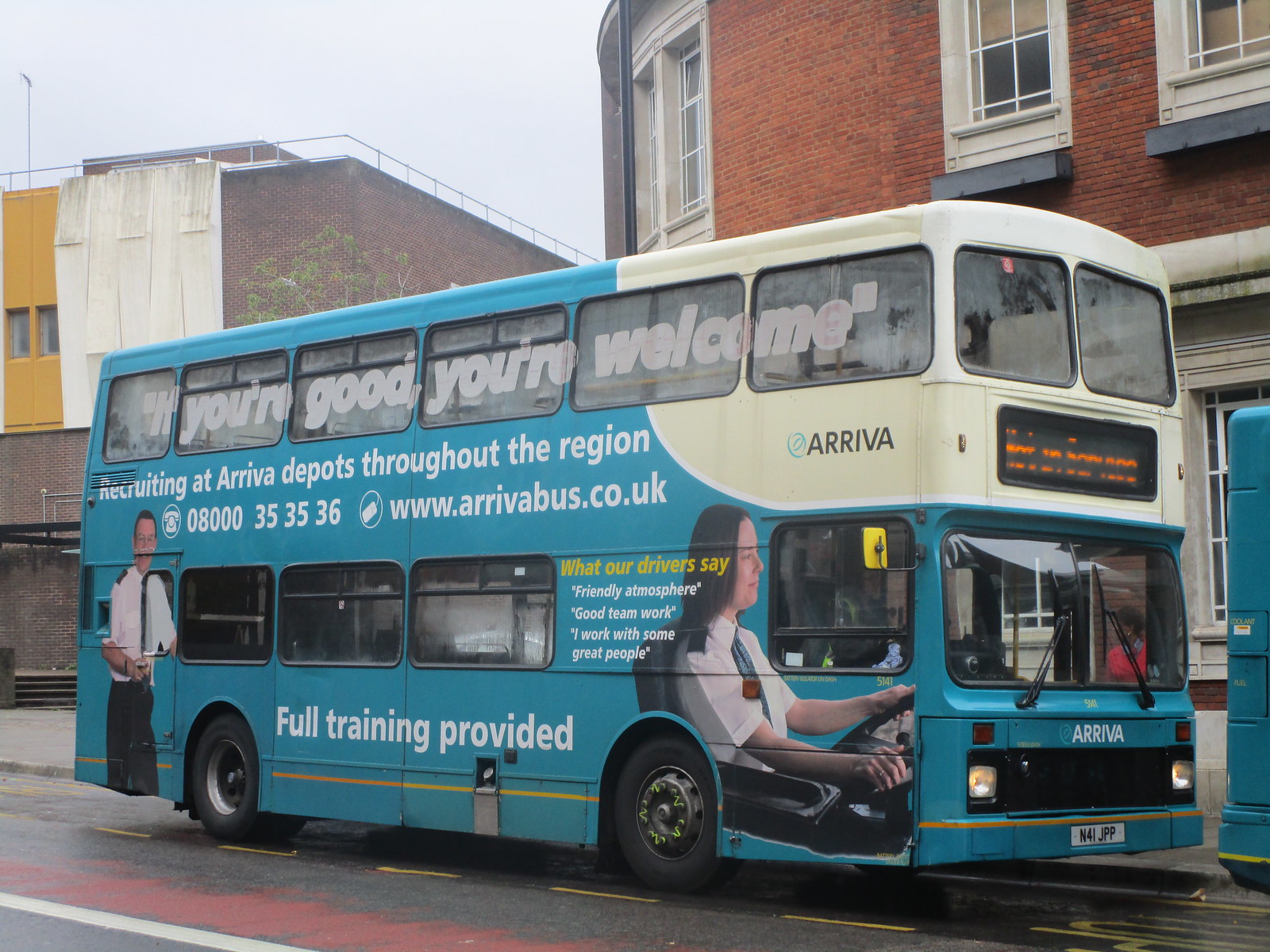The photograph showcases a light blue double-decker bus adorned with a large recruitment advertisement for Arriva. The bold white and gold text promotes job opportunities at Arriva depots throughout the region, emphasizing "Full training provided." The tagline, "If you're good, you're welcome," is prominently displayed across the top windows of the bus. The bus features visuals of two cheerful employees: a woman behind the wheel and a man smiling at the camera. Additionally, the ad highlights testimonials from drivers praising the friendly atmosphere and good teamwork at Arriva. The bus is parked in an urban environment, flanked by large buildings—one characterized by red brick and white windows, and the other by white and yellow elements with guardrails atop. The sky overhead is gray, adding a typical UK backdrop, further confirmed by the website www.arrivabus.co.uk. Despite the bus's information screen being partially obscured and unreadable, the overall promotion is vivid and informative, aiming to attract potential recruits.